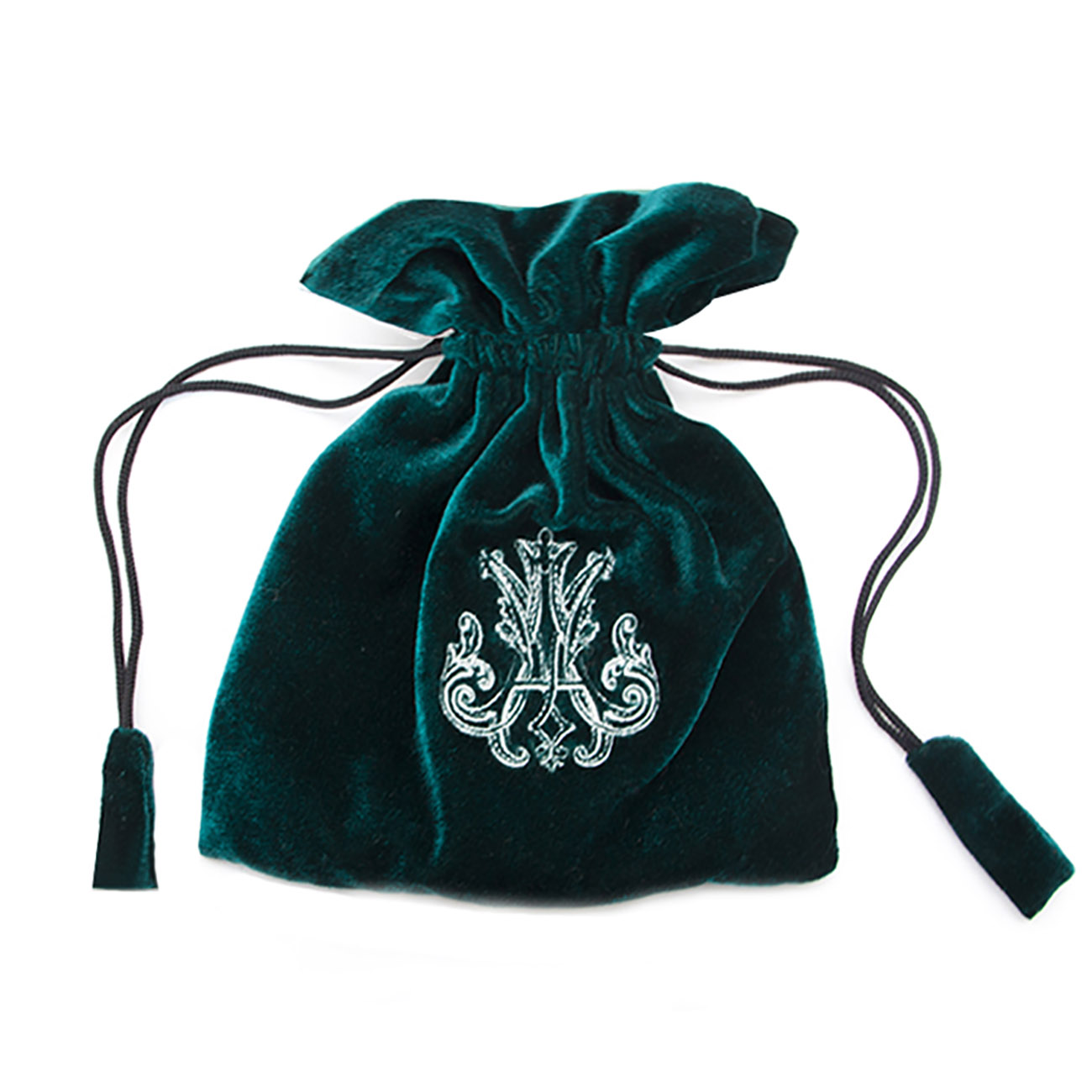The image features a small, dark green velvet drawstring pouch with two cords, one extending from each side. The luxurious fabric exudes a soft and gentle texture, reminiscent of suede or velvet, making it pleasing to the touch. The cords, equipped with matching green pulls, allow the pouch to be securely closed. Centered on the front of the pouch is an abstract design, possibly resembling the letter 'A', rendered in solid white. This design occupies approximately 20-30% of the pouch's surface area. The pouch, while small in size—suggesting it could hold items like dice for D&D, perfume vials, or serve as a renaissance cosplay accessory—stands out against the stark white background of the image, enhancing its intricate details and rich color.